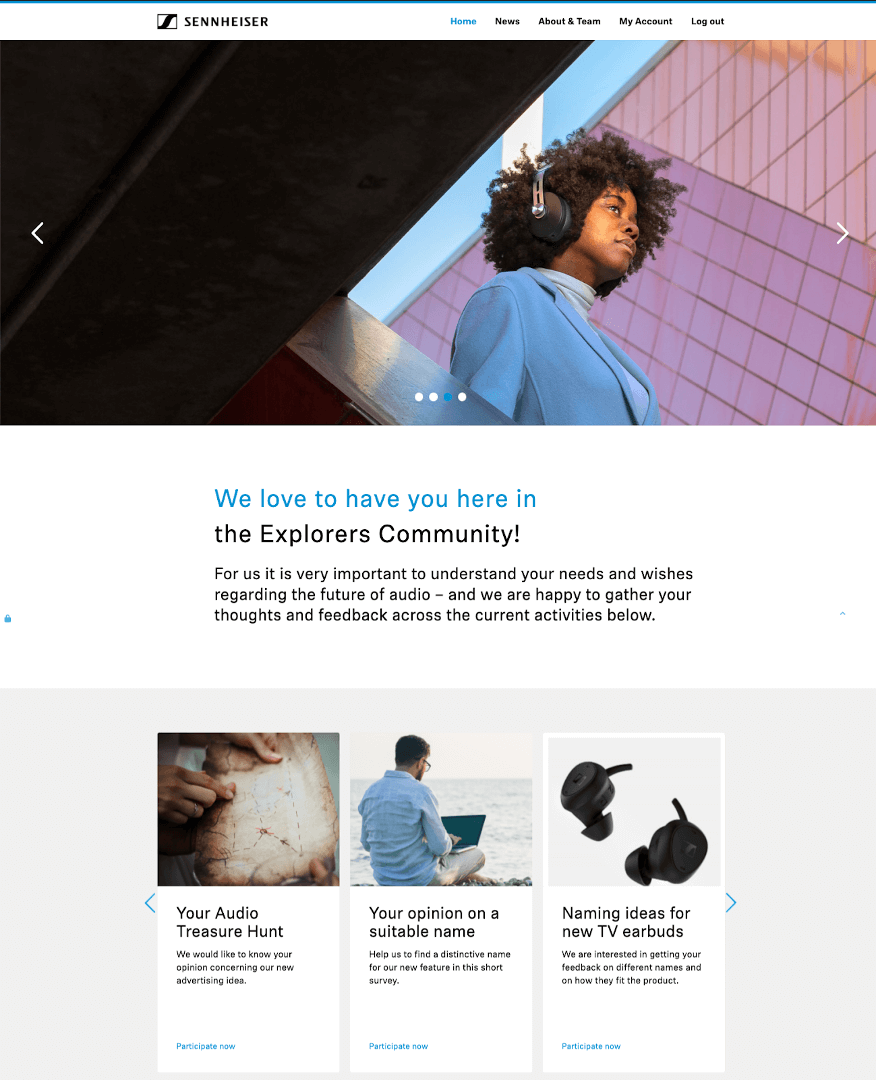The image is a detailed screenshot from a website. At the top, there's a thin, bright medium-blue line. Directly below it, there's a white banner which contains a prominent square on the left-hand side with bold, thick text reading "SENNHEISER" in all capital letters.

Moving horizontally from left to right, there is a navigation menu consisting of the following options: "Home" in blue text, followed by "News," "About," "Team," "My Account," and "Logout." 

Beneath the menu, there's a large graphic depicting an individual walking by buildings while wearing over-the-head headphones. Below this graphic, on a white background with some off-white elements, there's blue text that reads, "We Love to Have You Here In." Following this phrase, in black text, are the words "Explorers Community," with the 'E' and 'C' capitalized. 

Further down, the background shifts to light-gray. This section is divided into three rectangular blocks, each featuring an image at the top and text at the bottom. The text in these blocks reads: "Your Audio Treasure Hunt," "Your Opinion on a Suitable Name," and "Name Ideas for New TV Earbuds," respectively.